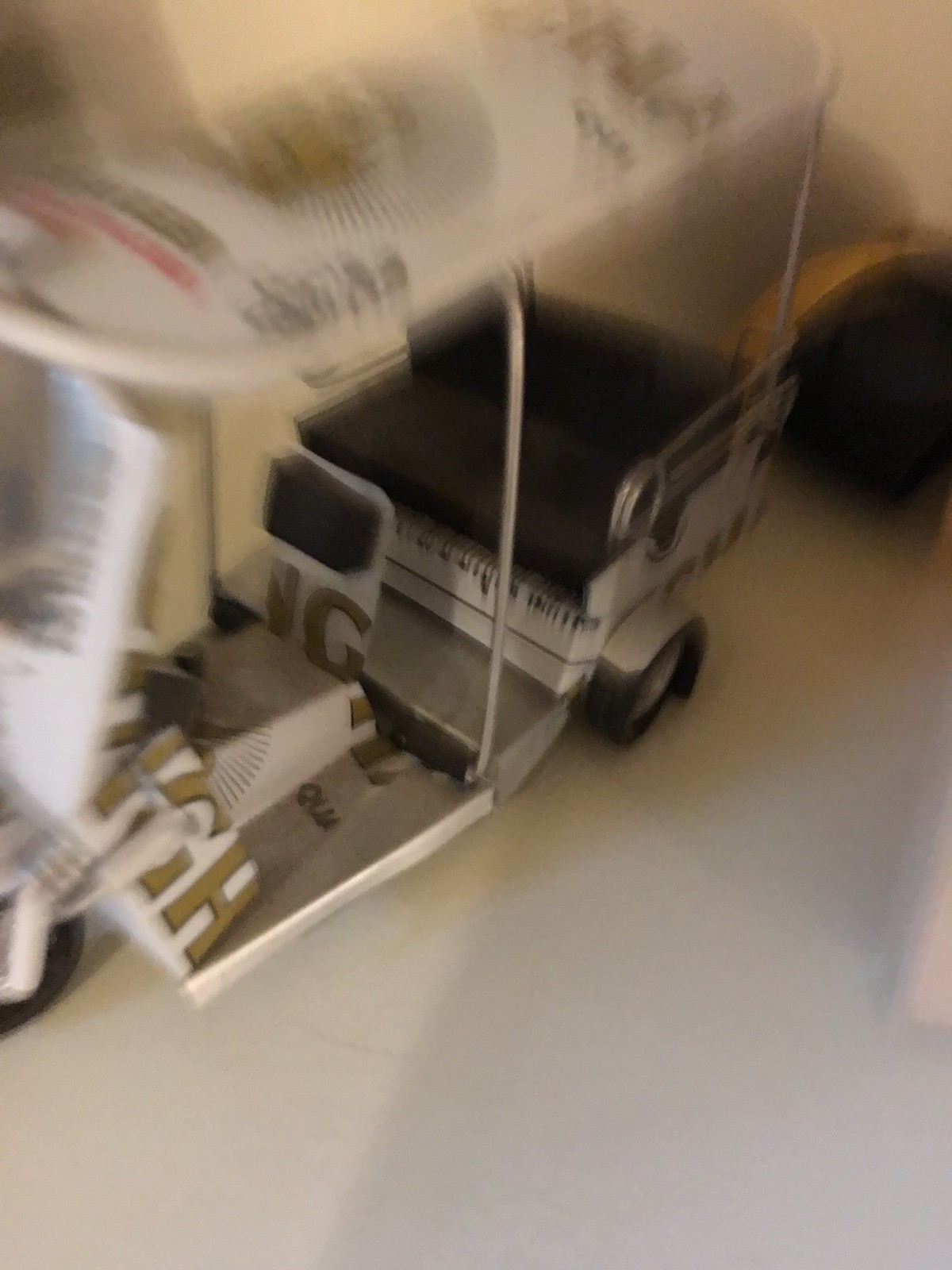The image features a unique three-wheeled golf cart that resembles a tricycle. The cart has a single seat positioned at the front center and a black back seat. Silver bars extend from the corners at the rear to the center, supporting a white roof adorned with gold letters and a gold symbol. Behind the cart, there is a gold arch and a black square, adding to the aesthetic appeal. The rear tire is partially covered by white fender covers, and a black cushion provides head support for the front seat. A white tube extends down to the front tire, contributing to the cart's distinctive design. The background of the image is white and somewhat blurry, focusing attention on the golf cart itself.